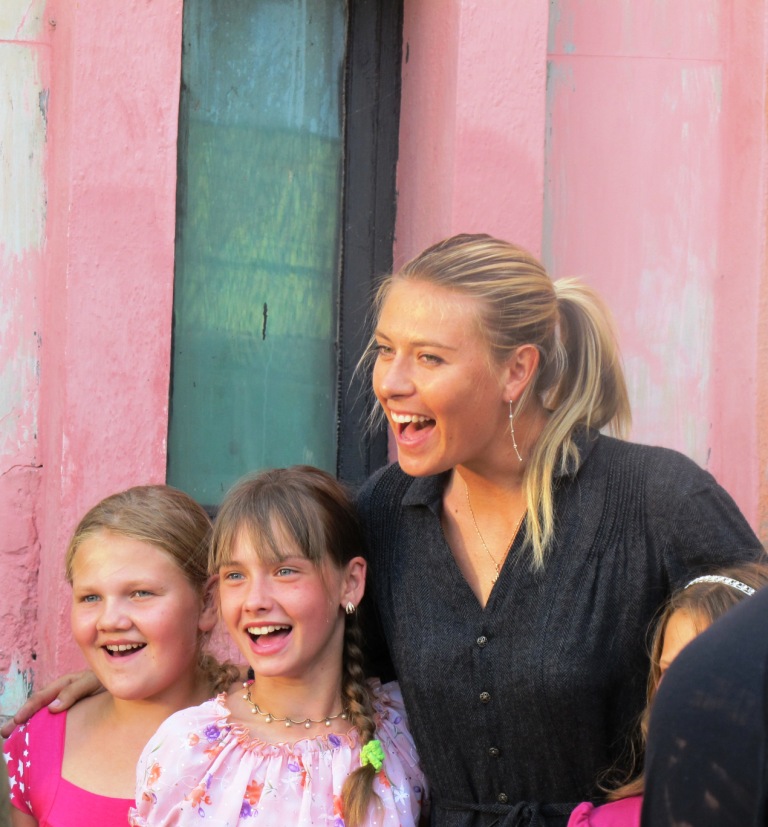The photograph captures a vibrant and joyful moment featuring a woman and three young girls. They are all posing and looking towards the bottom left corner of the image. The backdrop is a weathered pink plaster wall with noticeable paint peeling off, revealing white and gray spots. A green support pillar stands prominently in the middle of this wall.

The central figure, an adult woman with dark hair streaked with blonde, has her hair styled in a ponytail and is adorned with long, rope-like earrings. She is dressed in a black, button-up shirt with a collar and a tie in the middle. Her mouth is open in a cheerful expression, showing the top row of her teeth. 

To the left of the woman stands a young girl with a braid draped over her shoulder. She wears a short-sleeved blouse adorned with a pink, purple, and white floral pattern and a small necklace. Next to her, another young girl with light brownish-blonde hair and light-colored eyes sports a round face and a pink, square-necked shirt. 

On the woman’s right, a young girl’s face is mostly obscured by another person's shoulder, but it can be seen that she is wearing a white, sparkly headband and a pink blouse. The edge of someone's elbow, dressed in a black shirt, can be seen in the bottom right corner, contributing to the joyful clutter of the group photo.